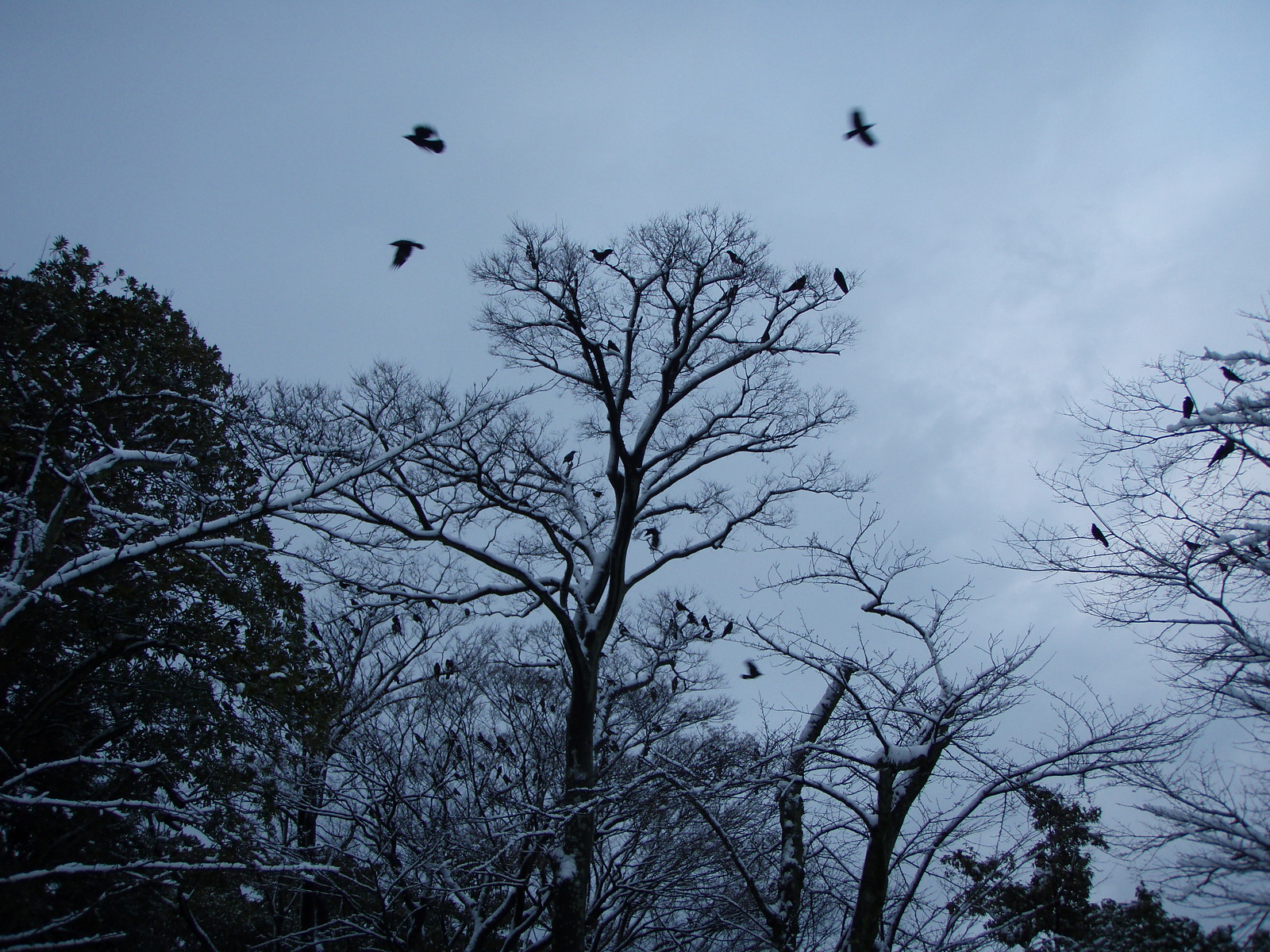This photograph captures an overcast, wintry scene just after sunset, bathed in a bluish-gray twilight. The sky is heavily clouded, seamlessly blending with the snow-covered ground. A row of trees lines the right and center parts of the image, most of them barren and covered in snow, their branches starkly silhouetted against the sky. On the left side stands a lone tree still adorned with snow-dusted leaves. Scattered throughout these trees and the sky are about twenty black birds, possibly crows. Some birds are perched on the branches, while several others are caught mid-flight, their motion creating a blurred effect. The entire composition exudes a cold, moody ambiance, accentuated by the soft blue tones that pervade the scene.